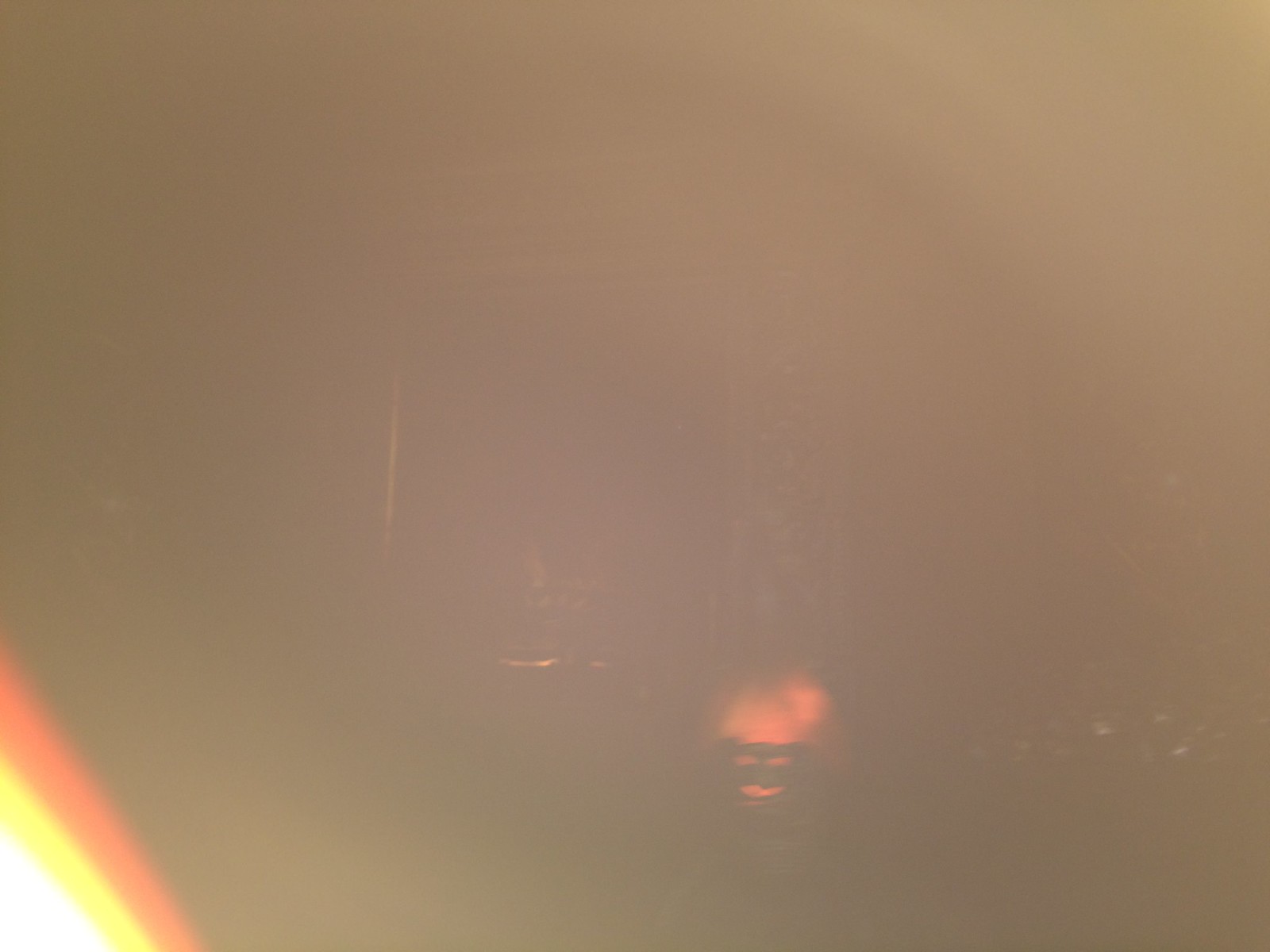In the image, a thick fog envelops the scene, casting a grayish hue over the entire area. On the left side, a bright white light pierces through the mist, transitioning into vivid yellow and red tones as it merges with the surrounding fog. The top right section of the scene also appears shrouded in gray.

At the center of the image, a fiery-red sphere or fire pit provides a striking focal point, its glow illuminating the surrounding area. Nearby, a speckled pillar stands alongside a bench, suggesting an outdoor setting. Overall, the composition hints at a misty, atmospheric environment with diverse light sources and a mixture of natural and man-made elements.